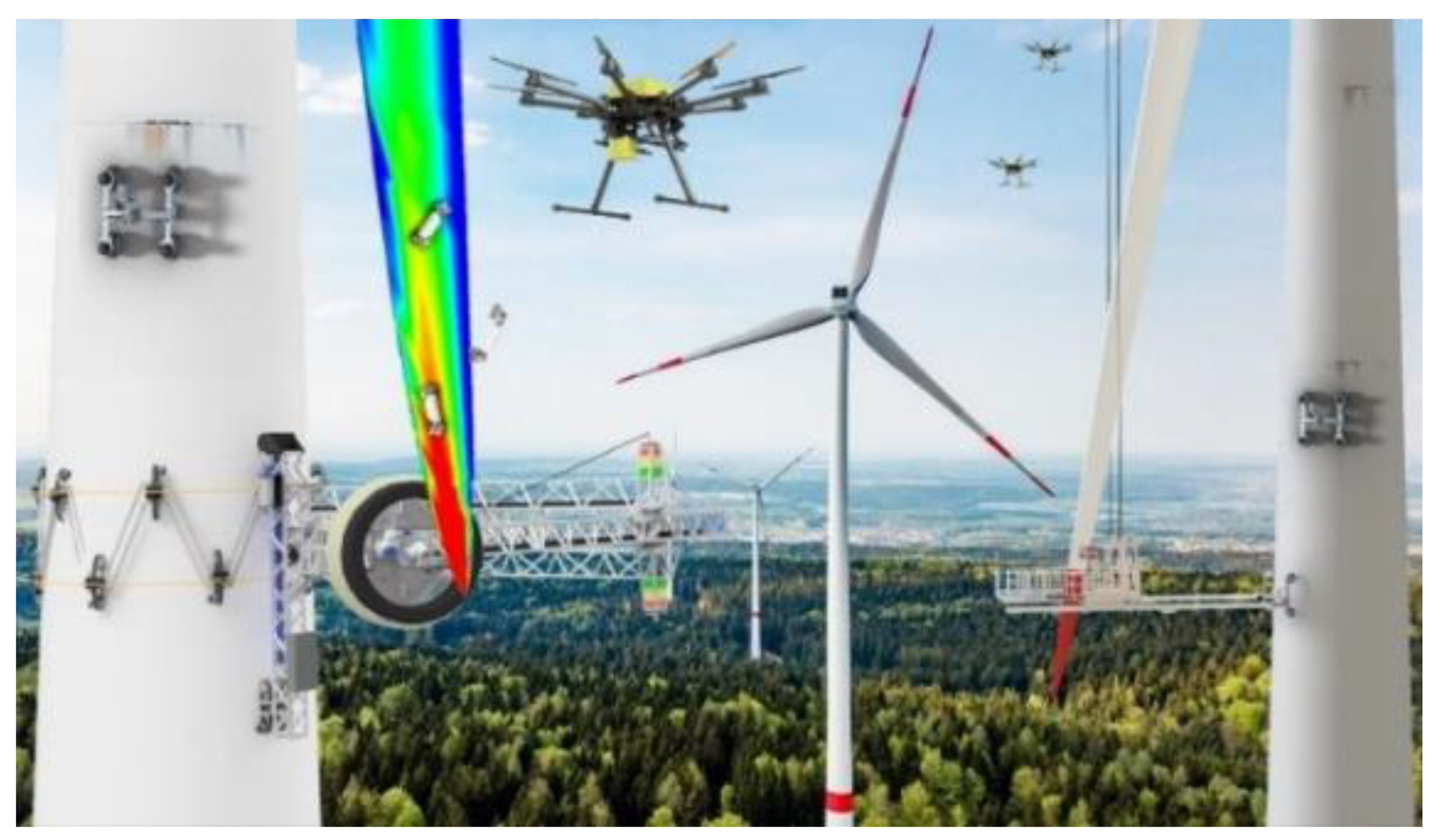This intricately edited digital image resembles a photo-realistic video game scene set in an outdoor daylight environment. The focal point features tall, modern white wind turbines adorned with rainbow colors emerging from the top, stretching from the bottom to the top. Numerous black and yellow drones are scattered throughout the bright blue sky with patches of clouds. The landscape below showcases a sprawling forest. The entire composition, a horizontal rectangle, also includes additional wind turbines in the distance, visible on both the left and right sides. These elements, juxtaposed with the serene background, contribute to a visually striking yet surreal image, giving it a unique, digitally manipulated appearance.